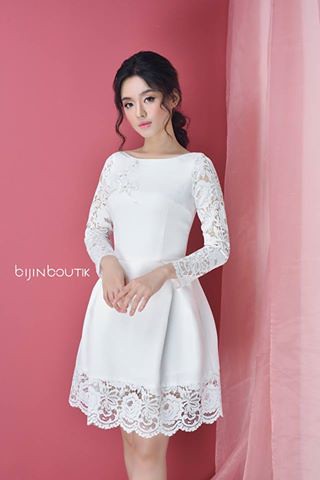The photograph features an Asian woman, or possibly of mixed ethnicity, posing in front of a pink wall with a transparent pale pink curtain draping down to her right. She has long, dark hair styled in a ponytail with two curled strands framing her face. The woman is dressed in a short, white cocktail or wedding dress that ends just above her knees. The dress boasts an open, wide-neck collar with see-through lace sleeves, and the bottom is adorned with a lace frill featuring a floral design. Her pale complexion contrasts elegantly with the vivid pink background. She gazes directly at the camera, likely serving as the model for an advertisement. To the right of her hands, near the middle of the image, the words "BIJIN BOUTIK" are visible, suggesting a promotional context for the dress she is showcasing.